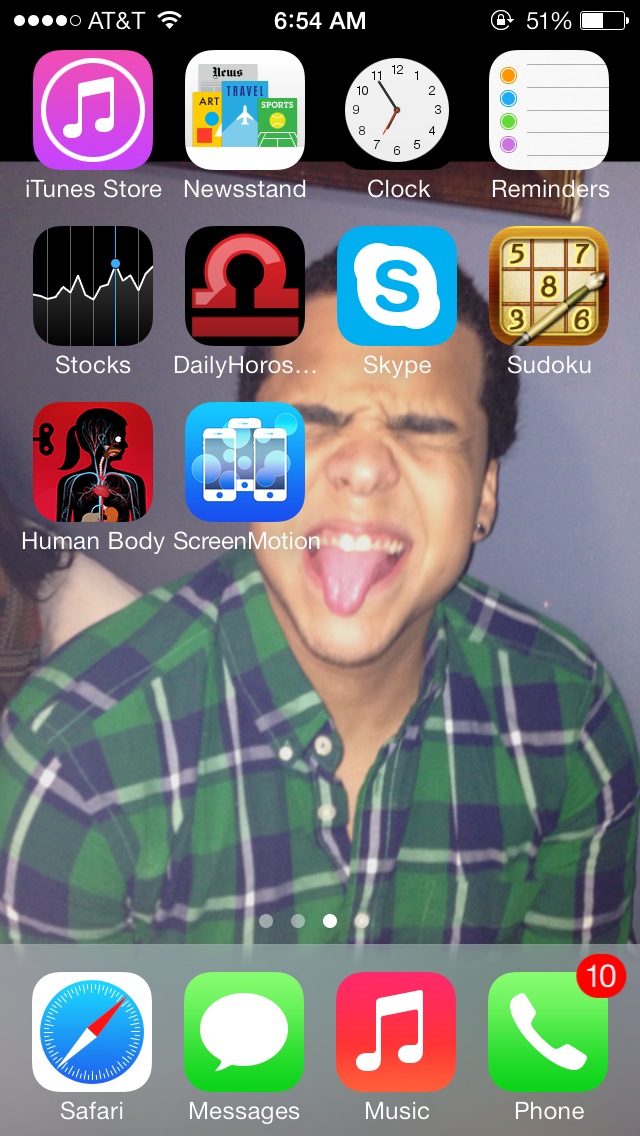This is a highly detailed screenshot of an Apple iPhone home screen. The top banner displays the time as 6:54 a.m. with a 51% battery life, flanked by TNT and Wi-Fi symbols on the left and right, respectively. There is a series of five dots, four white and one black, indicating different screen pages. The background features a man with dark hair wearing a green and blue plaid shirt with white stripes, eyes closed, and sticking his tongue out. The middle to bottom of the screen shows the wallpaper image partially obscured by various app icons. Listed apps include iTunes Store, Newsstand, Clock, Reminders, Stocks, Daily Horoscope, Skype, Sudoku, Human Body, and Screen Motion. At the bottom of the screen are four dock icons for Safari, Messenger, Music, and Phone, the latter showing 10 missed calls. The color palette on the screen includes purple, pink, green, blue, yellow, black, white, red, brown, tan, and orange, making for a vibrant and detailed display.